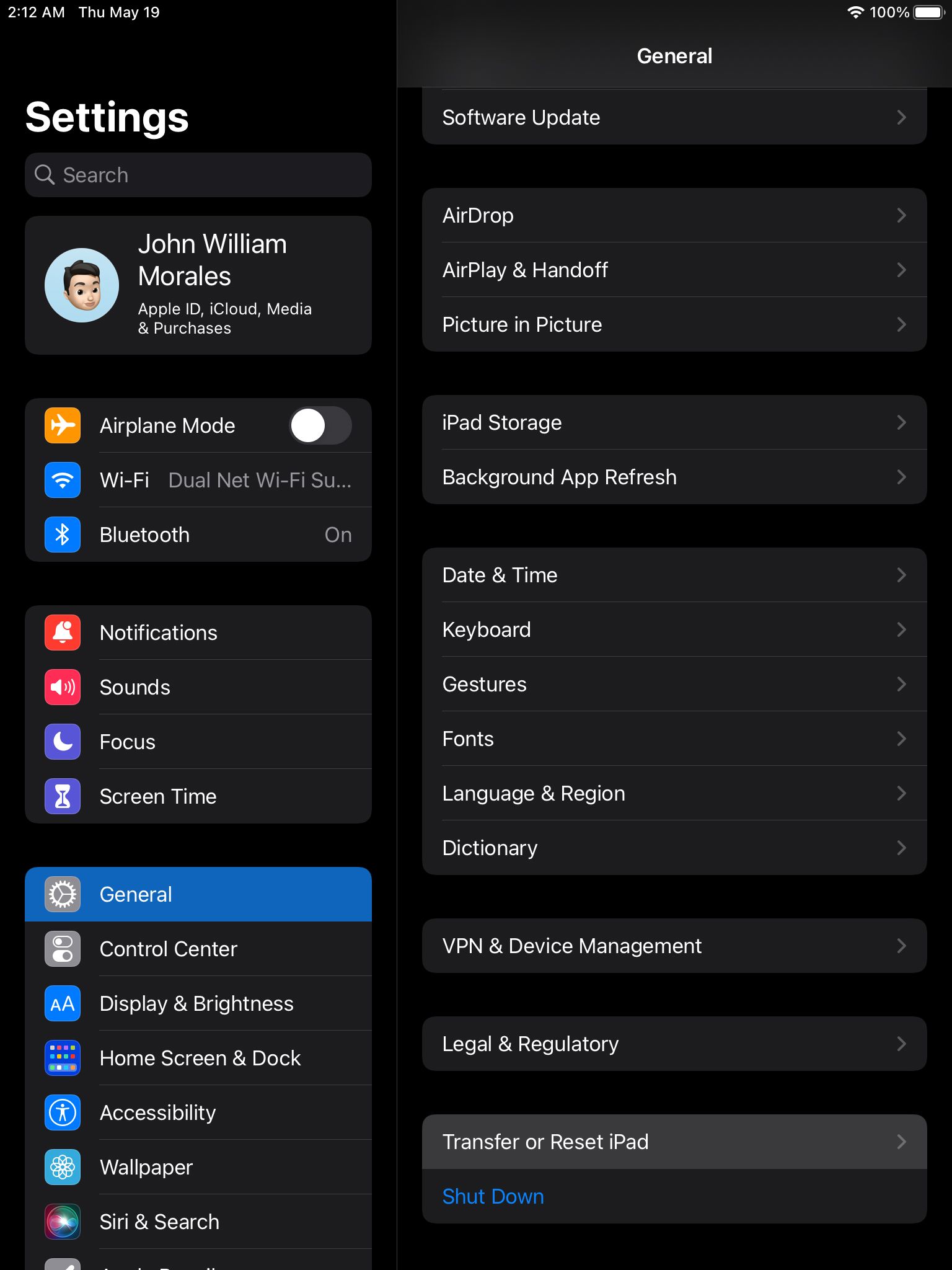Screenshot of a mobile device's settings interface in dark mode.

In the top left corner, the current time is displayed as 2:12 a.m., Thursday, May 19th. The top right corner shows the battery at 100% and a fully engaged Wi-Fi signal.

The background is black, while the menus are rendered in a charcoal gray, indicative of dark mode. On the left side, there's a vertical menu. At the top, in white font, it states "Settings." Below this, there's a search field with a white magnifying glass icon. Underneath, it displays "John Williams Morales - Apple ID, iCloud, iTunes & App Store," accompanied by a cartoon icon of a man's head with brown hair.

The first listed option is "Airplane Mode," with an adjacent airplane icon, which is toggled off. Next is "Wi-Fi," showing a connection to "DualNet Wi-Fi…." 

Following that, "Bluetooth" is toggled on. Subsequent options include "Notifications," "Sounds," "Focus," "Screen Time," "General," "Control Center," and "Display & Brightness."